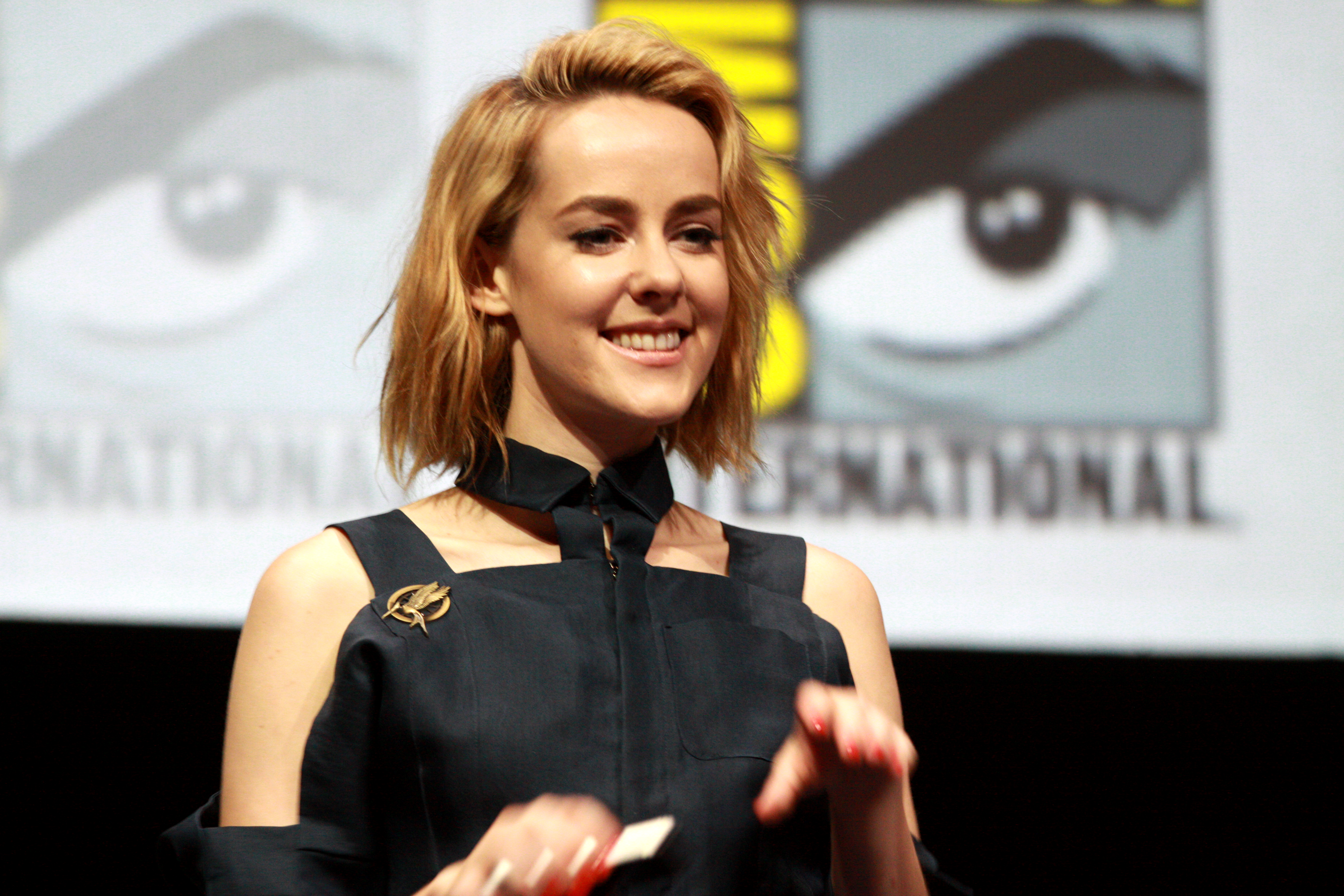This photograph captures a woman who closely resembles Kristen Stewart, smiling and engaging in conversation at the Comic-Con International event. Her dark blonde hair, styled in a shaggy bob, falls just above her shoulders. She is wearing a distinctive black outfit featuring a halter-style top with straps that accentuate her bare shoulders, and a shrug or shawl that covers her arms down to the elbows. Her nails are painted a dark orange, and her hands appear blurred, suggesting movement. She embellishes her ensemble with a prominent gold pin on her upper left chest, depicting a circular design with a hummingbird or Mockingjay emblem, indicating a possible promotion related to "The Hunger Games." The backdrop features the recognizable Comic-Con International logo, partially visible with its yellow letters and a cartoon eye emblem on a white background above a black banner. The overall ambiance suggests she is actively engaged and enjoying the event.